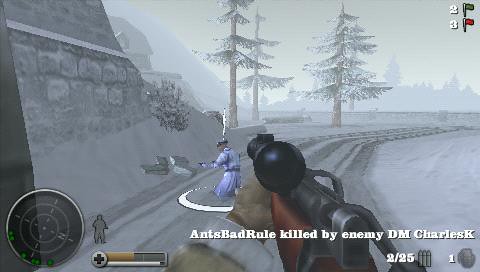In this screenshot from a first-person shooter video game, the player’s character is seen holding a gun pointed at an enemy lying on the snowy ground. The wintry landscape features numerous snow-covered trees, adding to the immersive environment. The in-game HUD (Heads-Up Display) reveals critical information: in the bottom right corner, text reads “Ants bad rule killed by enemy DM Charles K,” possibly indicating a recent in-game event or kill. The player's ammunition count is displayed, showing 2 out of 25 bullets and a single available grenade. At the top of the screen, two flags represent team scores—gray with a score of 2 and red with a score of 3. The bottom left corner hosts a health bar and a stamina meter, along with a miniature map indicating the positions of enemy players. The overall scene suggests an intense moment of gameplay in a competitive, team-based shooter setting.